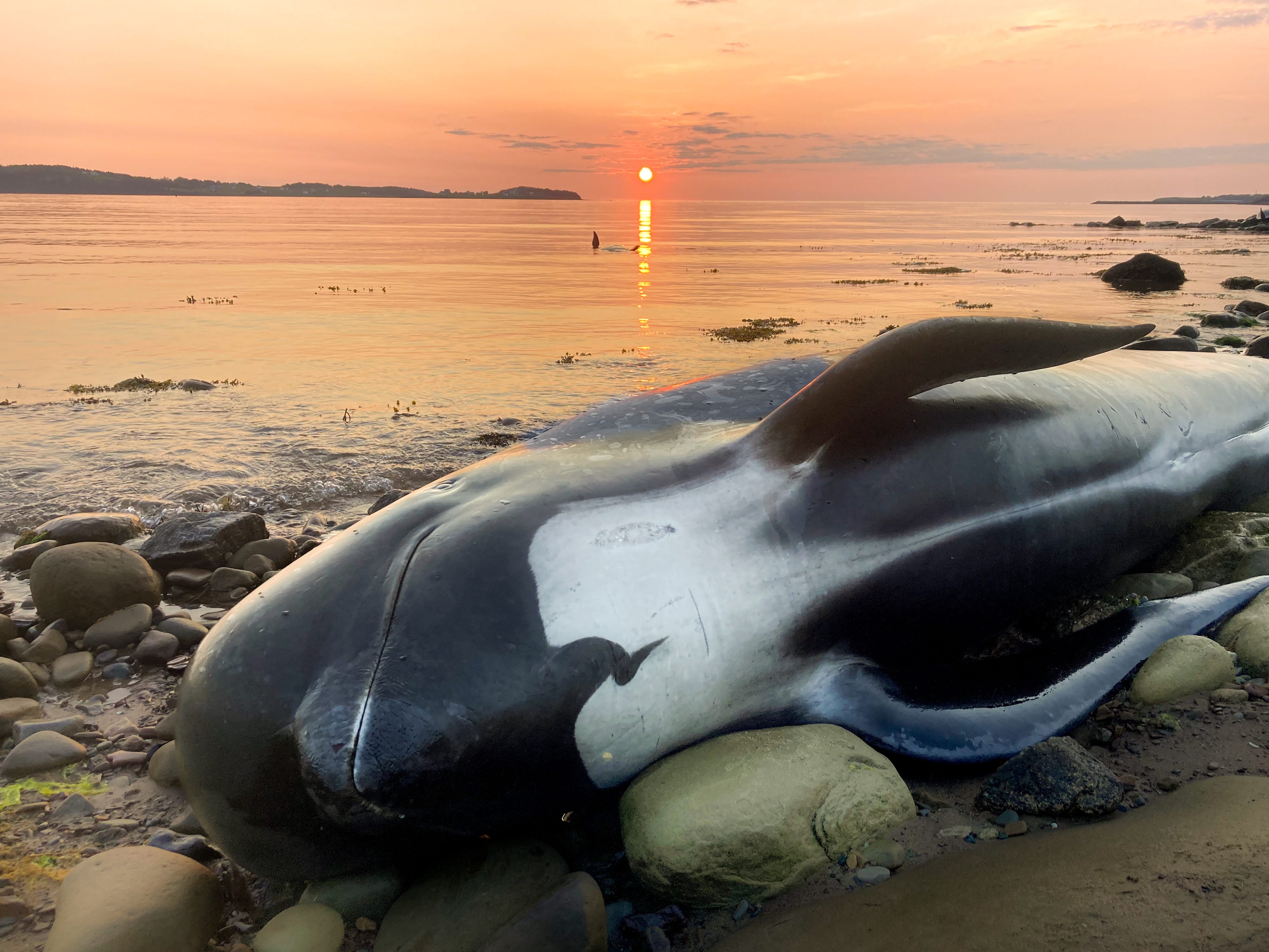A haunting yet striking photograph captures a deceased black and white whale beached on a rocky shoreline at sunset. The whale lies on its side, its black head, back, fins, and belly contrasted by a white neck area, sprawled out on the brown and gray rocks. The desolate scene shows the effects of the tide, with water seemingly receding to reveal a sandbar. Surrounding the whale, scattered rocks and stretches of somber brown dirt heighten the melancholy. In the far background, the setting sun casts a warm glow across the ocean's surface, with brilliant hues of orange, yellow, pink, purple, and lavender painting the sky and reflecting gently on the water. Majestic hills or mountains loom on the horizon under the radiant, orange sun, capturing a moment of poignant beauty and sorrow.